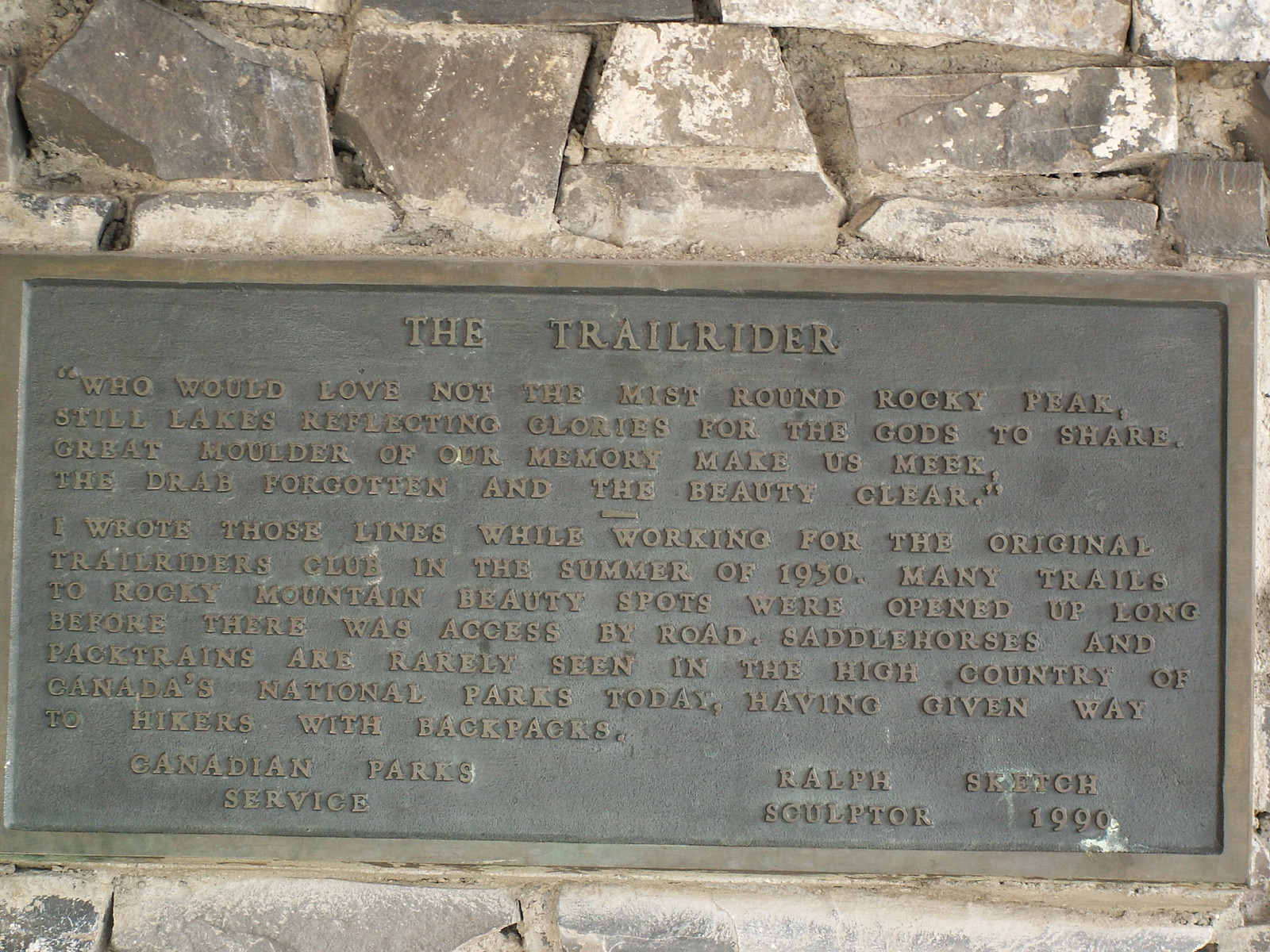This color photograph, likely taken outdoors during the daytime, captures a historical marker affixed to a rugged rock wall. The wall consists of loosely assembled chunks of gray and black rock, showcasing patches of white with no visible mortar. The metal plaque, adorned with raised embossed lettering, bears the title "The Trail Rider." The plaque includes poetic lines: "Who would love not the mist round rocky peak, still lakes reflecting glories for the gods to share. Great moulder of our memory, make us meek, the drab forgotten and the beauty clear." Below, it reveals a narrative from 1930, detailing the author's experience working for the original Trail Riders Club and how many trails to Rocky Mountain beauty spots were established long before the advent of road access. Today, the sight of saddle horses and pack trains in Canada's National Parks has mostly been replaced by hikers with backpacks. The marker, dated 1990 and credited to Ralph Sketch as Sculptor, is a testament to this historical transition facilitated by the Canadian Park Service.